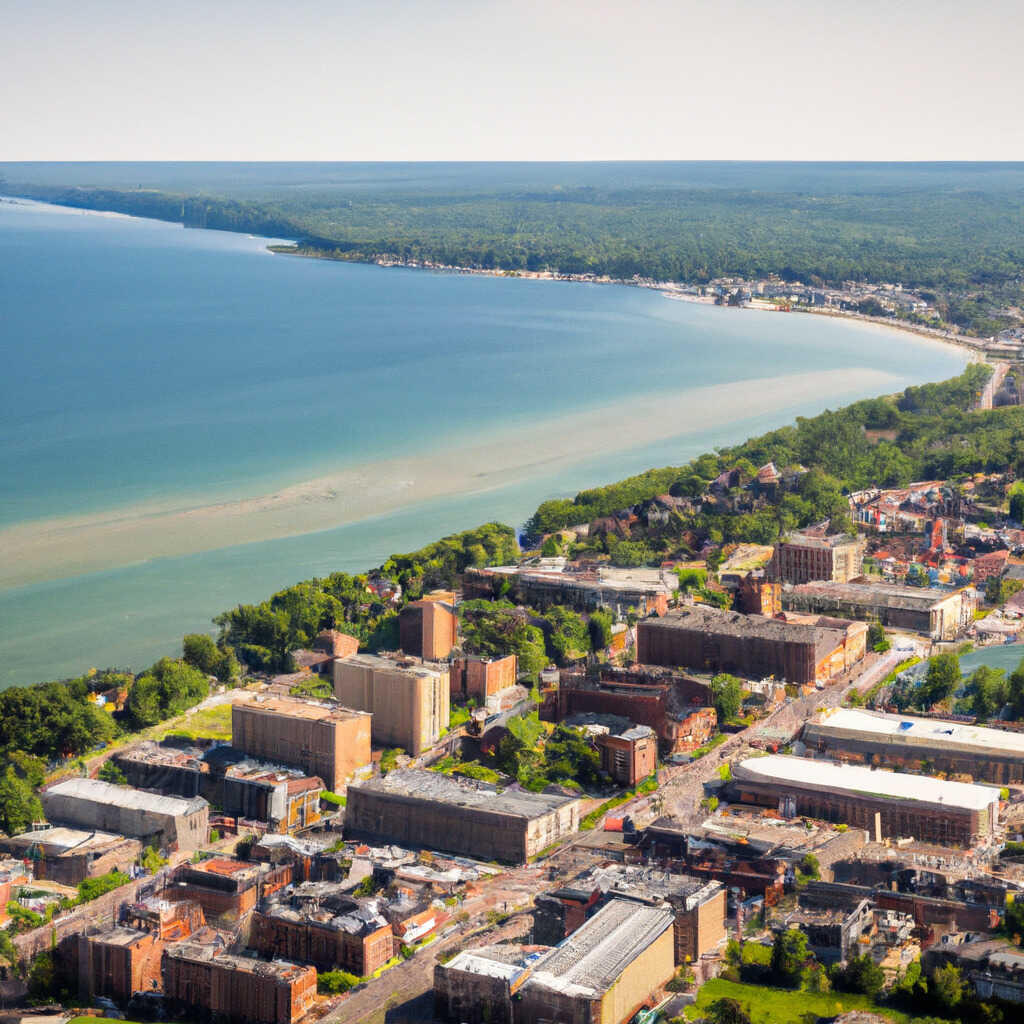An aerial photo captures a sprawling shoreline that forms an angular corner, starting from the bottom left, progressing upward to the top right, and making a bend back towards the left. The central beach transitions through shades of blue, turquoise, and green as it nears the sandy shore, dotted with tree-lined areas and a notable sandbar just offshore. Dominating the lower portion of the image, a cluster of industrial-looking rectangular and square buildings in hues of cream, tan, and brown appears unflattering against the scenic backdrop. The midsection has a bustling walkway or leveled incline densely populated with people. Extending towards the top right, more houses and a slender beach line emerge among a sea of verdant trees. Far off into the distance, the shoreline townscape blends into a horizon of continuous green canopies, under a blanket of light gray, overcast skies. While a main street traverses the town's center, the image's pixelation obscures finer details such as vehicles. Overall, this lively and complex coastal scene reflects a small town rich with natural and constructed elements.